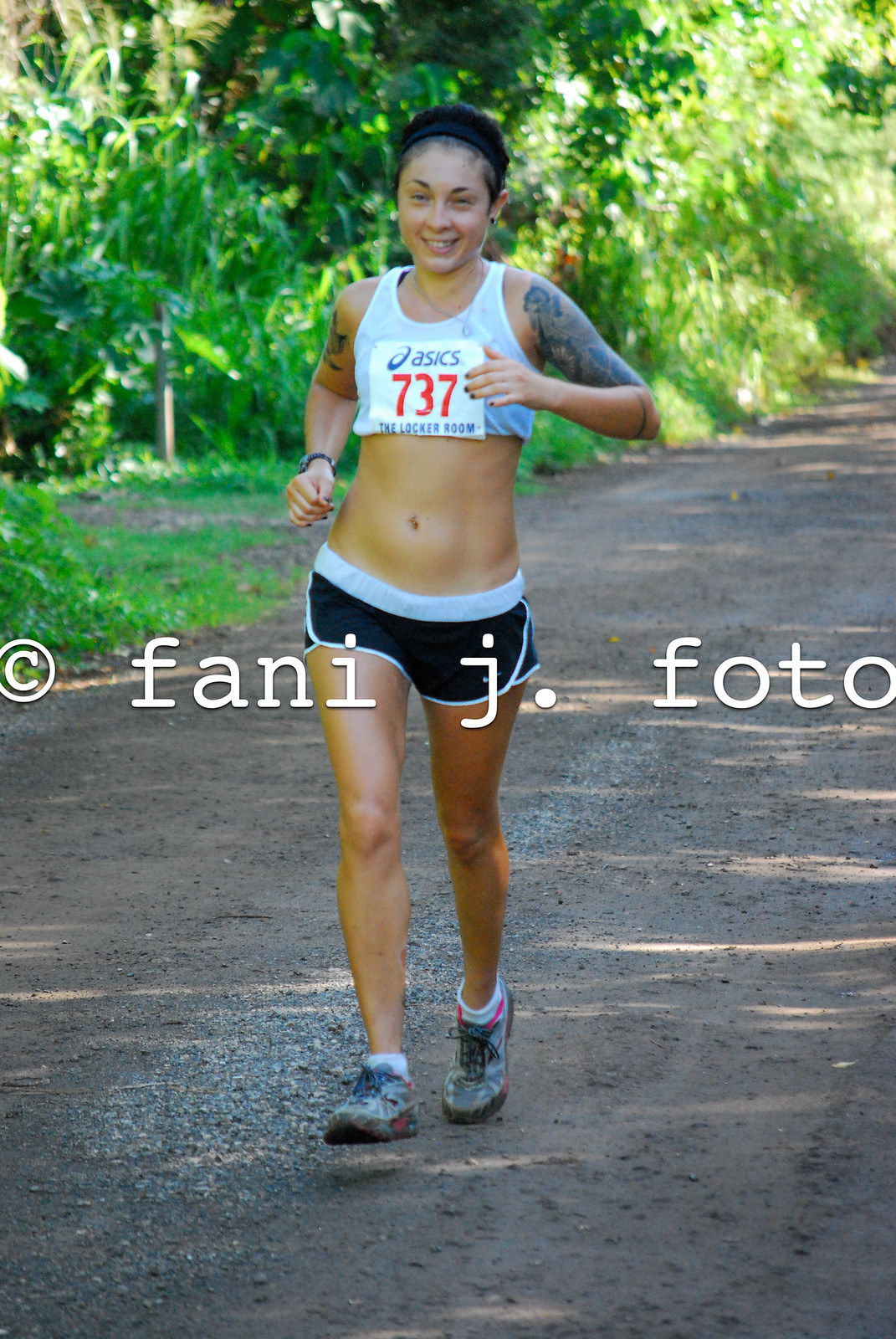In this photo, a determined runner with black hair, held back by a wide black band, is captured mid-stride during a marathon on a dark, dirt or gravel road. Her attire, consisting of a very short white tank top rolled up to expose her midriff and deep blue or black shorts with a white waistband and piping, suggests the hot weather she is enduring. She is identifiable by her race bib, which prominently displays the ASICS logo, the number 737 in red, and "the locker room" written below it. Adorning her left wrist is a wristwatch, and her body features extensive tattoos: one fully covering her left arm and a smaller one on her right arm. The dense greenery of the background contrasts sharply with her outfit and the road, indicating a lush, perhaps forested, environment. A significant watermark on the image credits Fanny J Photo, ensuring the copyrighted work is recognized.